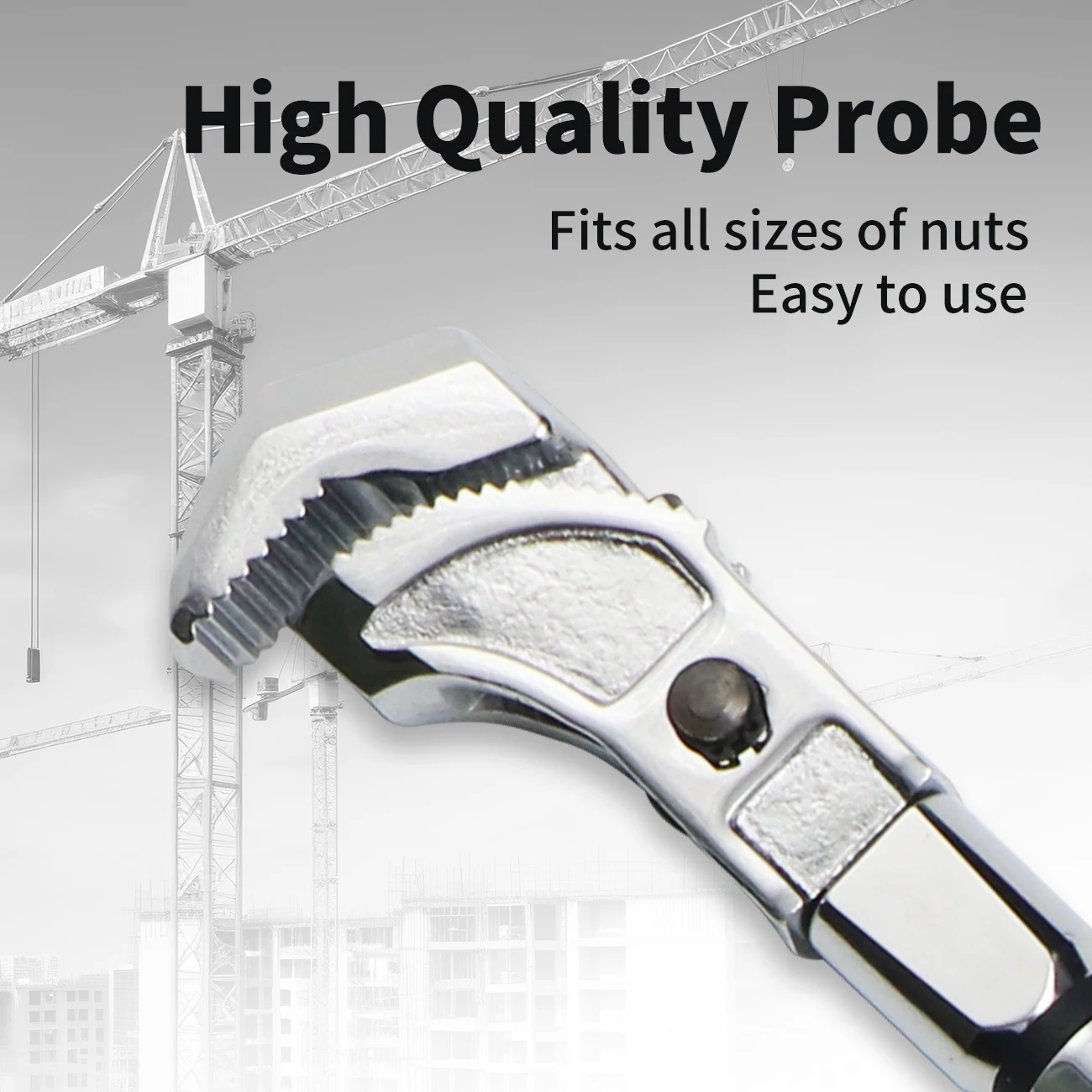The black and white advertisement features prominently displayed text at the top reading "High Quality Probe" in bold black letters, followed by the phrases "fits all sizes of nuts" and "easy to use" in a slightly smaller, non-bolded font. Below this text, the central focus is an enlarged, highly detailed photograph of a silvery metal wrench with a chrome finish. The wrench includes a distinct black knob on its side and visible metal teeth at the top. Notably, the wrench exhibits varying textures, with a shiny base and a more textured middle. The background consists of a black and white image of a construction site, featuring buildings at the bottom and a tall crane to the left, indicative of the tool's utility in construction settings.